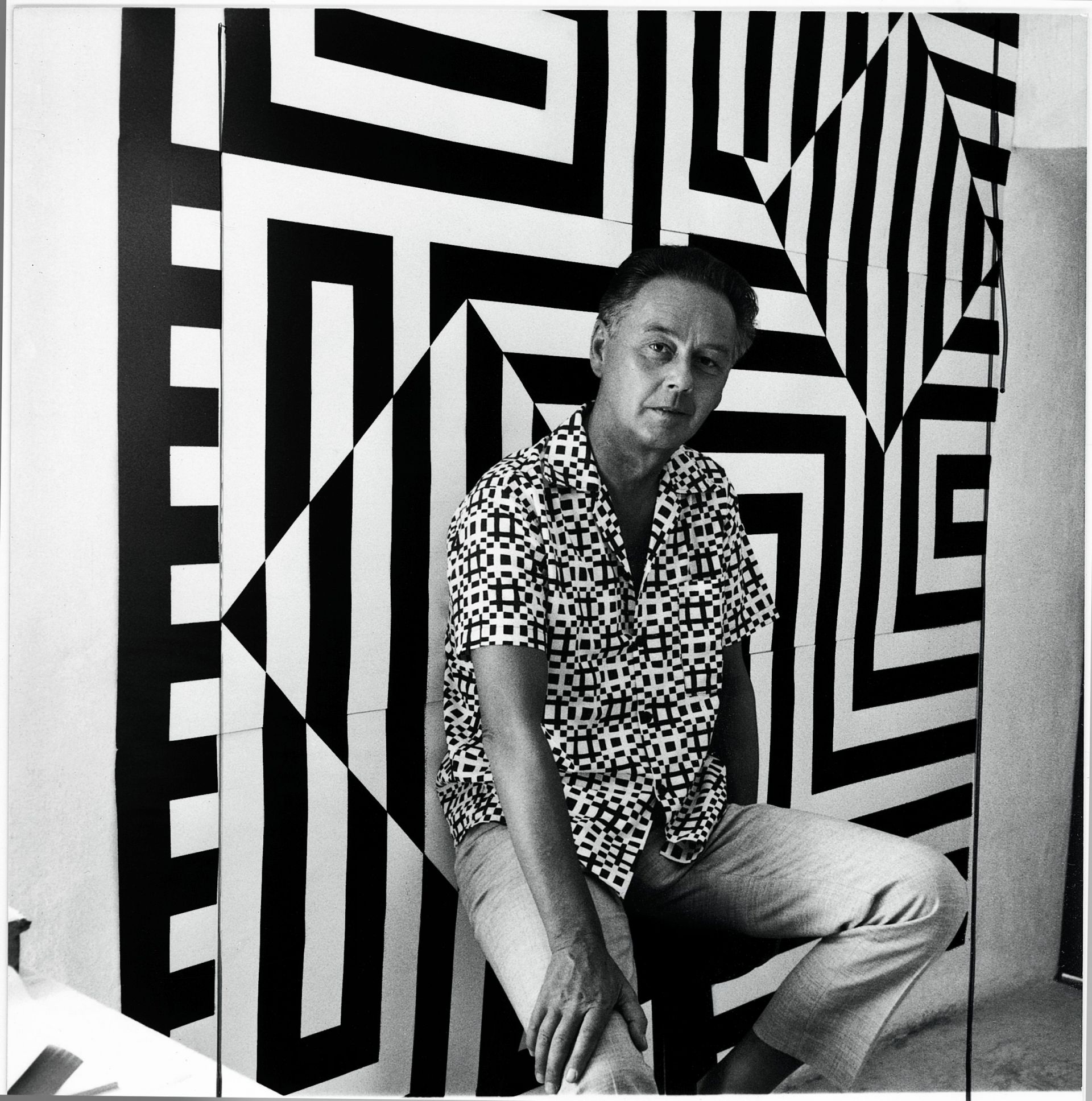This black-and-white photograph features a middle-aged man seated on a dark-colored stool positioned slightly to the right in the image. The man, who has short, dark hair with grey at the sides, wears a short-sleeved, open-collared shirt adorned with black and white geometric designs that mirror the bold patterns in the background. His light-colored linen pants contribute to a casual yet coordinated look. He is facing the camera, with his left hand resting beside his left leg and his right hand placed on his right knee. The backdrop consists of a striking black-and-white mural filled with various geometric figures such as oblongs, diamonds, and squares, with lines crisscrossing in different directions. This mural is flanked by sections of white stucco wall. Additionally, a small table with indiscernible items is visible on the left side of the image. The ground beneath his stool appears to be carpeted.